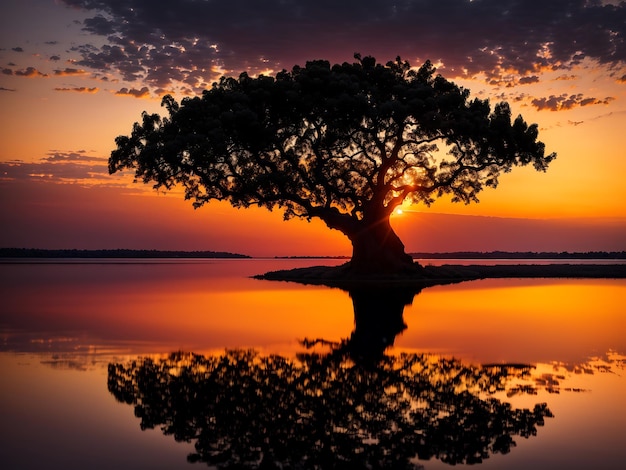A stunning sunset scene features a large, wide tree with a thick, short trunk and expansive branches fanning out like a Japanese maple, silhouetted starkly against the vibrant sky. The tree stands at the center of a calm lake, its dark reflection mirrored perfectly on the still water. The colors of the scene transition dramatically from deep oranges and yellows near the horizon to purplish grays in the clouds above. The sun, setting behind the tree, casts an ethereal orange glow, highlighting the peacefulness and tranquility of the moment. The water's surface is entirely smooth, capturing the mesmerizing contrast between the bold silhouette of the tree and the vivid, reflective sky.